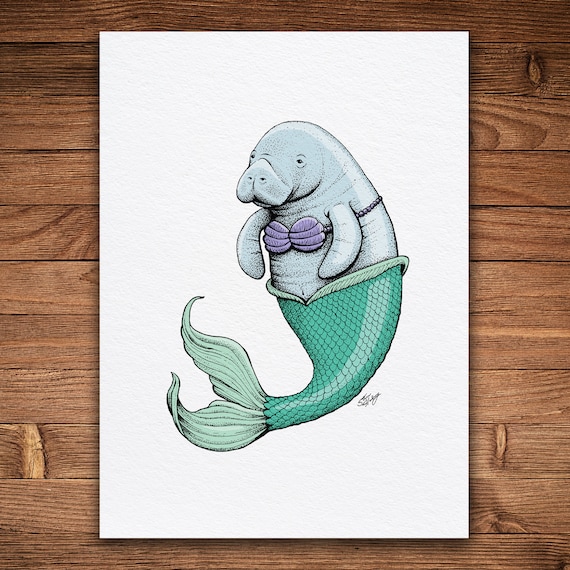The photograph captures a whimsical pen and ink drawing, displayed on a brown wooden table. The subject of the drawing is a unique mermaid-walrus hybrid. The creature features an aqua-scaled mermaid tail and a light grayish-white walrus upper body, adorned with a purple seashell bikini top. The walrus, which appears to be female, is gazing directly ahead, creating an engaging connection with the viewer. The drawing, vividly rendered in color, is on an 8 1⁄2 by 11-inch white piece of paper. A signature follows the curve of the tail, marking the artist's identity. The detailed and imaginative artwork stands out on the wooden surface, characterized by its playful and unusual concept.